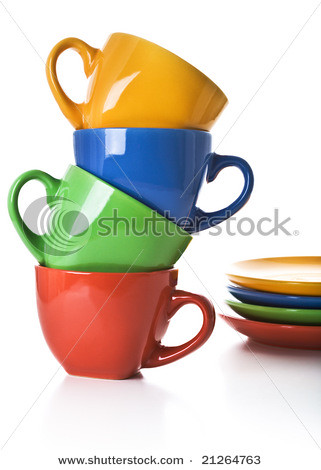This vertical stock image, watermarked with "Shutterstock" in a transparent gray font, features a close-up of four stacked ceramic coffee mugs and their matching saucers, all against a clean white background. At the bottom of the image, it reads "www.shutterstock.com" followed by the number "212-647-63" in small black font. The mugs, stacked one inside the other at slight angles, display a vibrant sequence of apple red at the bottom, bright green, blue, and a deep yellow at the top, with their handles pointing in alternating directions. To the right and slightly towards the rear, matching saucers are partially visible, stacked in the same color order with only their left halves shown. The white tabletop and minimalistic background emphasize the vivid colors and glossy ceramic texture of the mugs and saucers.